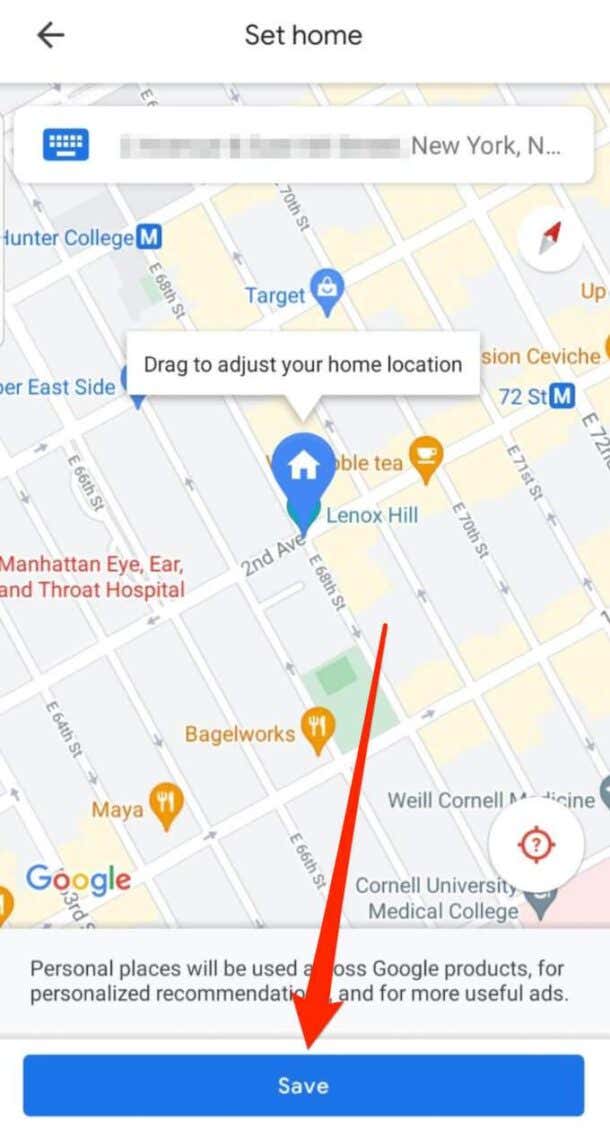This is a detailed screenshot of Google Maps on an iPhone, depicting the setup process for defining a home location. At the top of the interface, there's a "Set Home" label next to a back arrow icon, indicating the iOS platform. Most of the screen is dominated by a map image showing the area around Cornell University Medical College in Manhattan, New York City. A search bar at the top of the screen displays the partially grayed-out search term "New York, New York." 

The focus of the screenshot is the process of setting a home location on Google Maps. A location marker icon, which features a circle with a house symbol, is positioned on the map. A pop-up message above the marker instructs the user to "Drag to adjust your home location." A prominent red arrow points downwards to a large blue "Save" button, guiding the user toward completing the setup. 

At the bottom of the map, a white bar contains a message: "Personal places will be used across Google products for personalized recommendations and more useful ads." This screenshot overall demonstrates the steps to configure a home address within the Google Maps application.